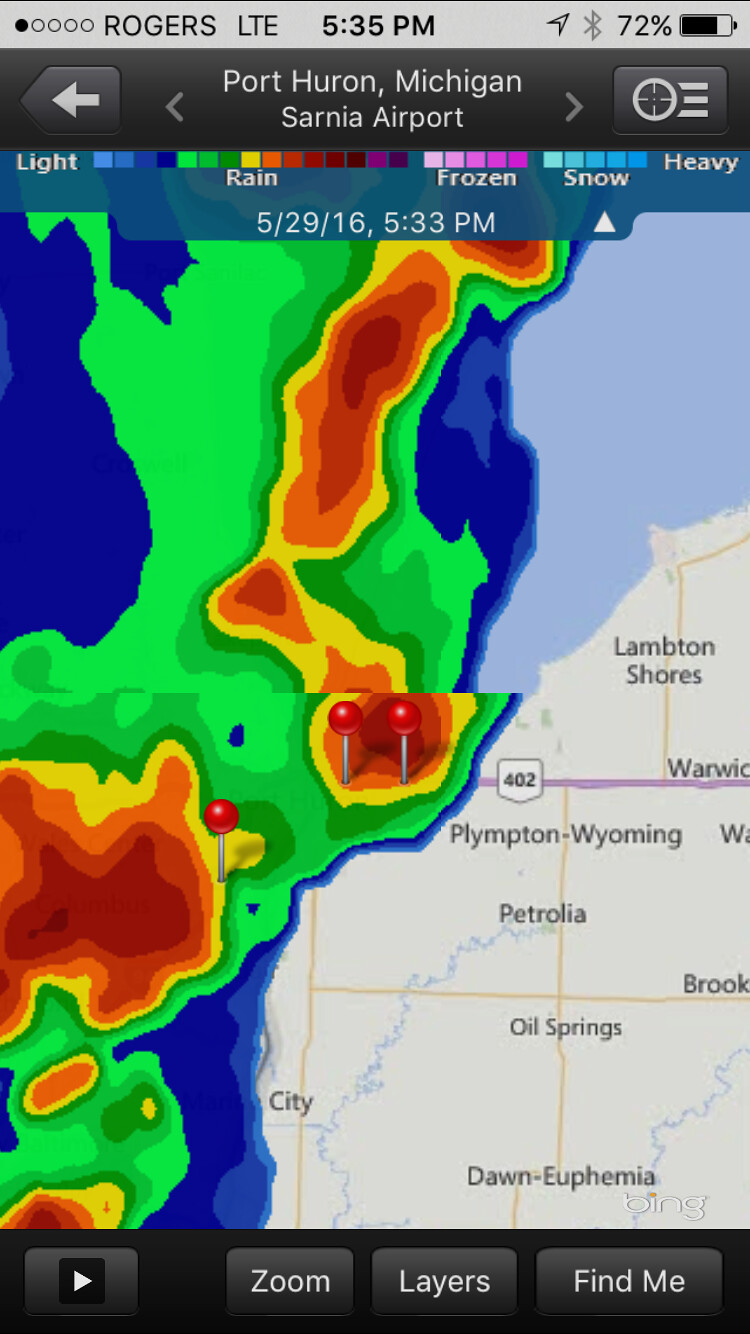This image appears to be a screenshot from a weather application on a mobile device. At the top of the screen, there is a gray horizontal bar showing network details "Rogers LTE," the time "5:35 PM," a Bluetooth icon, and a battery indicator at "72%." Below this bar, another strip displays navigation options with arrows, and the heading "Port Huron, Michigan, Sarnia Airport." The central part of the screen showcases a detailed weather map depicting precipitation intensity through a spectrum of colors: light green for light rain, scaling up to dark red for heavy rain. Several cities are marked on the map, including Petrolia, Oil Springs, Plumton, and Wyoming, along with freeway number "402." A color legend at the top explains the map's color codes ranging from light blue to dark red, indicating varying precipitation levels like rain and snow. At the bottom of the screen, there is a dark horizontal bar with interactive buttons labeled "Zoom," "Layers," and "Find Me." The map itself features a mix of dark blue, green, orange, and red shades, showing different precipitation intensities, and is complemented by street lines and city names for better location context.